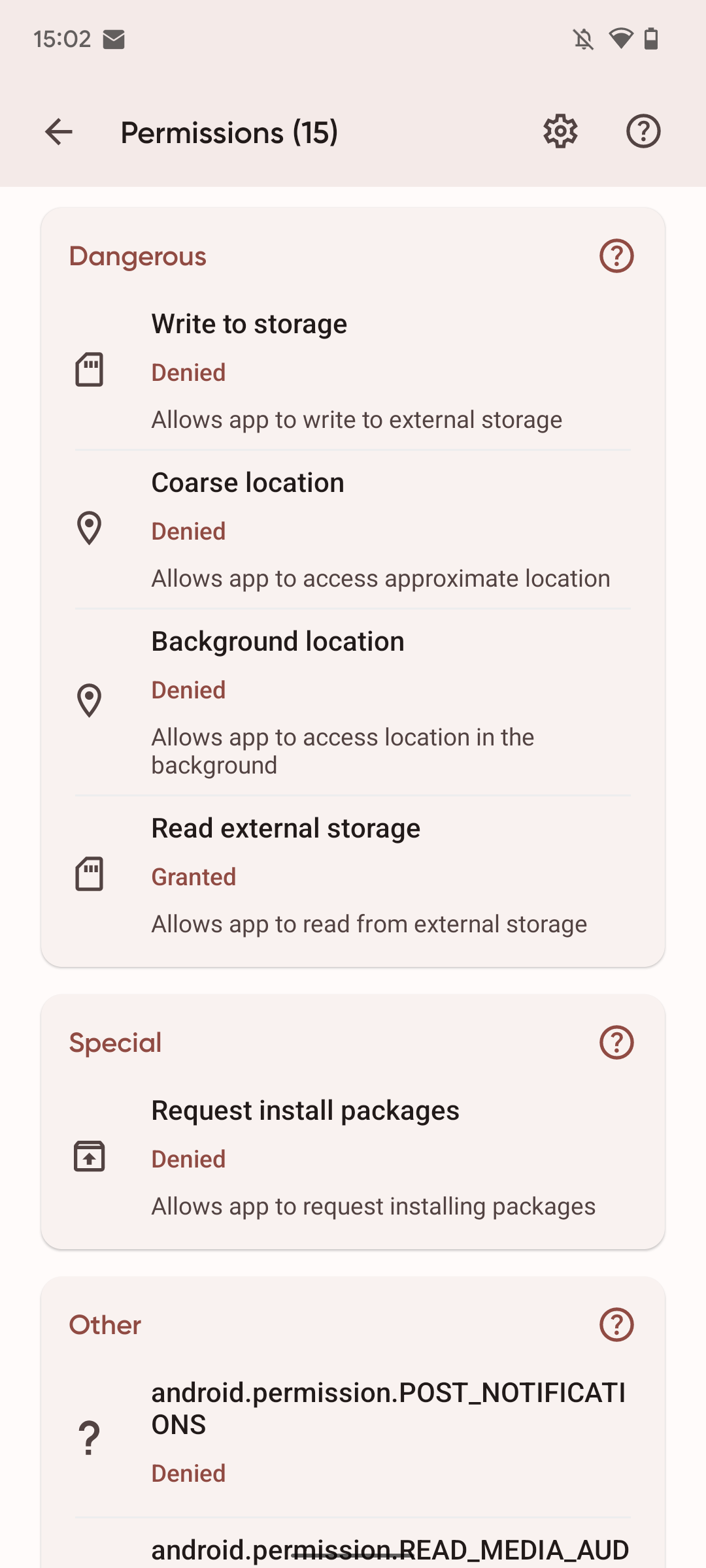This image is a detailed screenshot of a settings page within a mobile application. The page features a pale pink header at the top, which contains several elements. On the top left, dark gray text displays "1502," next to an email icon. Positioned on the top right are three additional icons.

Towards the bottom left of the header, a dark gray left-pointing arrow is followed by black text that reads "Permissions" with "16" in parentheses. On the right side of the header, after some negative space, there is a dark gray cog icon followed by a dark gray question mark icon encased in a circle outline.

Beneath the header lies the main body of the page, set against an even lighter pink background. The content is arranged into three primary rectangular sections, each with rounded corners.

The first section begins with red text reading "Dangerous" in the top left and a red question mark at the top right. Within this section, permissions are displayed in well-defined rows, each divided by thin light gray lines that almost stretch across the entire width. Each permission has an accompanying icon to the left, a black title slightly up and to the right, a red status next to it, and a light gray description beneath the status.

From top to bottom, the permissions are listed as follows:
- "Write to Storage": Denied, with a description reading "Allows app to write to external storage," paired with an SD card icon on the left.
- "Course Location": Denied, with a description stating "Allows app to access approximate location," accompanied by a geolocation pin icon.
- "Background Location": Denied, with a description noting "Allows app to access location in the background," indicated with another geolocation pin icon.
- "Read External Storage": Granted, with a description saying "Allows app to read from external storage," and an SD card icon to the right.

Two more sections follow this, each separated from one another by a thin area of the lighter pink background.